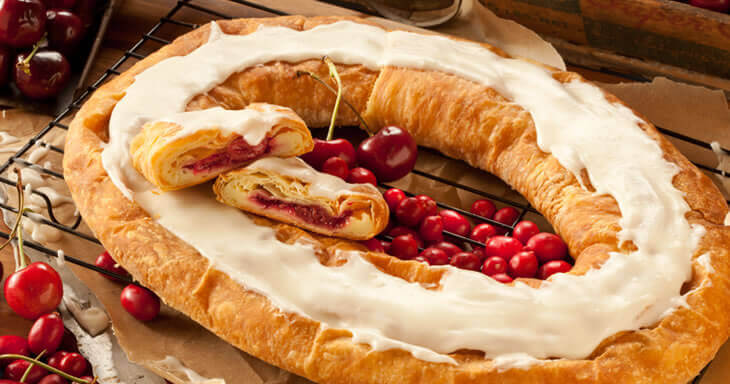A vibrant color photograph captures a delectable ring-shaped pastry, showcasing its light golden-brown crust. The pastry is circular with an open center, topped with a generous layer of white frosting forming a thick ring around its outer edge. Intriguing toppings are set within the ring, including two plump red cherries with their stems artfully crossed to form an X. Also placed atop the pastry are two slices taken from a different pastry, revealing the interior’s flaky multi-layer crust filled with luscious red jam, confirming that this pastry remains whole. The pastry itself rests on a black wire baking rack, visible through the open center. Adding an extra touch of color and freshness to the scene, scattered cherries are visible in the top left and right corners of the image.